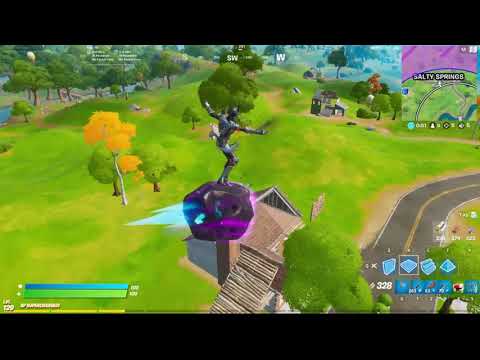This detailed screenshot captures an active moment in a video game, likely Fortnite. Central to the image is a character in a superhuman costume, poised mid-air while balancing on a purple rock or meteor with a blue flame emitting from its back. The character stands with arms outstretched as if flapping wings and has one leg kicked forward, suggesting dynamic movement. Surrounding the character is a lush, grassy landscape interspersed with various trees, including a prominent birch tree on the left with a white trunk and orange leaves. The backdrop features multiple pathways, a two-lane road on the right, and several houses. At the upper right corner of the screen is a mini-map displaying the text "Salty Springs," while at the bottom left, a health bar and a mana bar are visible in green and blue, respectively. The bottom right corner displays building materials such as staircases and pyramid shapes, alongside the number 328. The vibrant colors in the image include greens, yellows, blues, purples, pinks, reds, and grays, adding to the cartoon-like aesthetic of this engaging game scene.